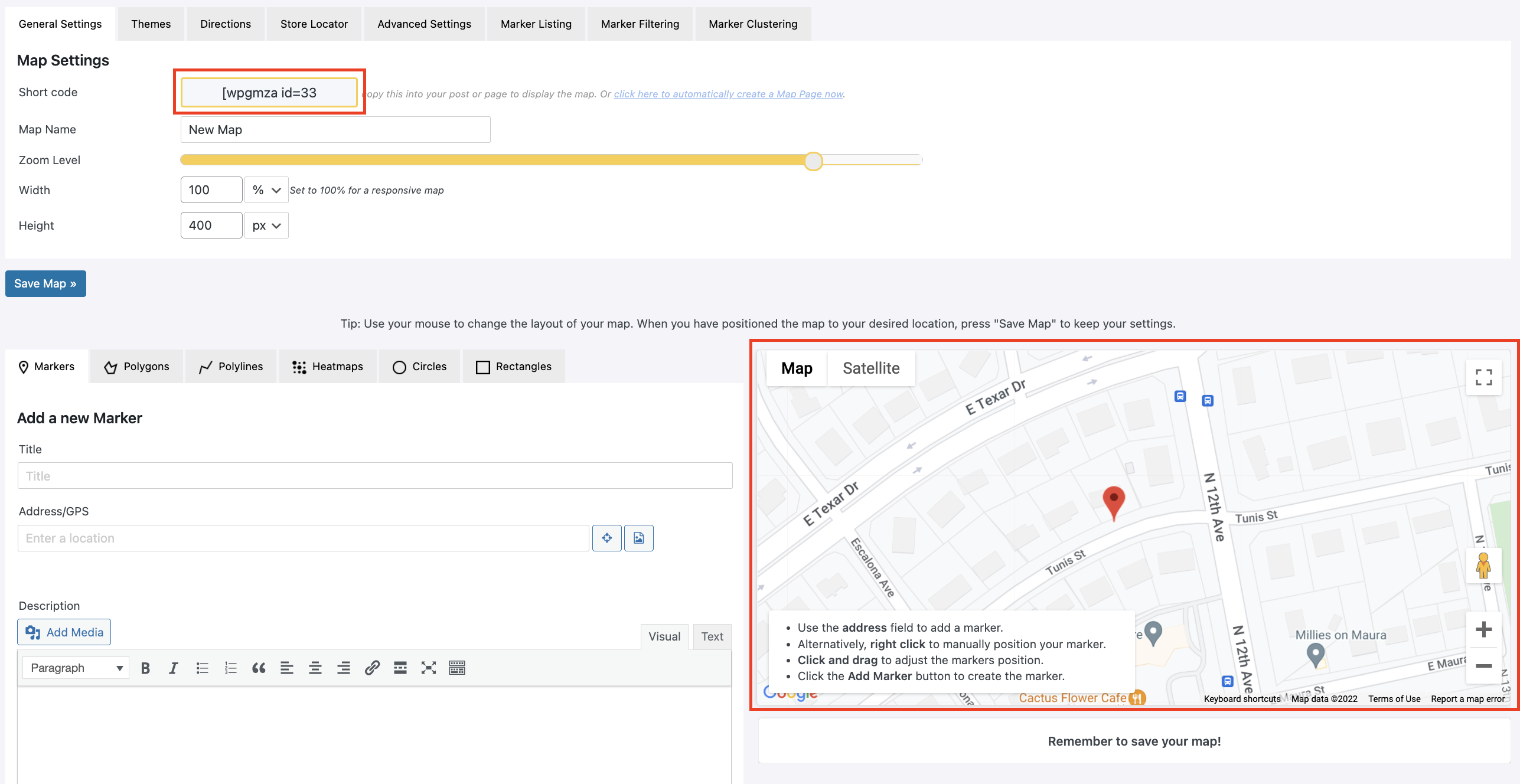The screen capture depicts a user interface, likely from a web-based map creation tool, set against a predominantly grayish-white background. At the top, a navigation bar includes black and gray submenu options such as "General Settings," "Theme," "Direction," "Store Locator," and "Advanced Settings." Beneath these main menus, sections labeled "Marker Listing," "Marker Filtering," and "Marker Clustering" are visible.

Further down, the interface displays a "Map Settings" area with black option names including "Shortcode," "Map Name," "Zoom Level," "Width," and "Height." Adjacent to these settings is a blue and white button labeled "Save Map." To the side, an orange and black box, highlighted in red-orange, contains a brief sentence in black and blue text.

Below, a white box labeled "Create New Map" is followed by a prominent gold bar with a gray circular icon. The interface features adjustable settings marked as "100%" and "400px," under a gray tooltip advising, "Use your mouse to change the layout of your map. When you've positioned the map to your desired location, press 'Save Map' to keep your settings."

Further elements include additional submenus for "Markers," "Polygons," "Circles," and "Rectangles," though the text is somewhat difficult to read. The section for adding a new marker provides fields for "Title," "Address," "GPS coordinates," "Description," and "Media," accompanied by a text box with various icons resembling those found in a word processor application.

The screen capture also shows a Google Map interface where users can switch between "Map" and "Satellite" views, with the "Map" view currently selected. A red box highlights this area, showing a red location pin and identifiable street names such as "Altex Dr." and "North 12th Avenue."

A black and white instructional box at the bottom guides users: "Use the address field to add a marker. Alternatively, right-click to manually position your marker. Click and drag to adjust the marker's position. Click the 'Add Marker' button to create the marker." Finally, a reminder at the bottom prompts users to save their map.